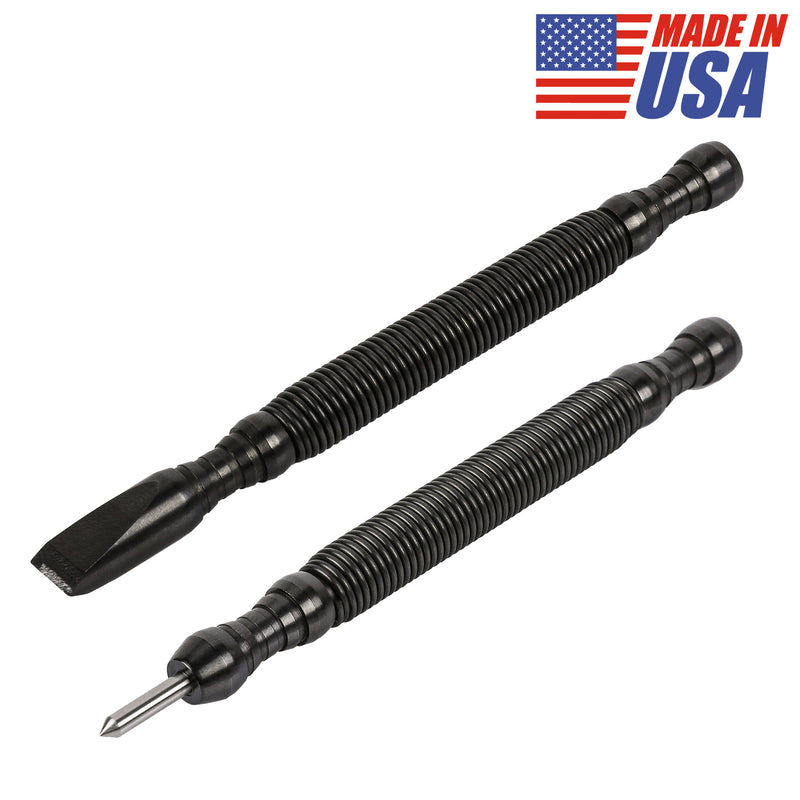Ad for a Winter Vehicle Toolset: Featuring a high-quality chisel and ice lock pick, both showcasing sturdy black handles and robust steel construction. Positioned with precision against a minimalist backdrop, these essential tools stand upright, emphasizing their reliability and craftsmanship. The upper right corner proudly displays an American flag, complemented by the bold text "Made in USA," with "Made in" rendered in striking red and "USA" in bold blue. This advertisement highlights indispensable tools designed to ensure your vehicle's safety and functionality during harsh winter conditions.